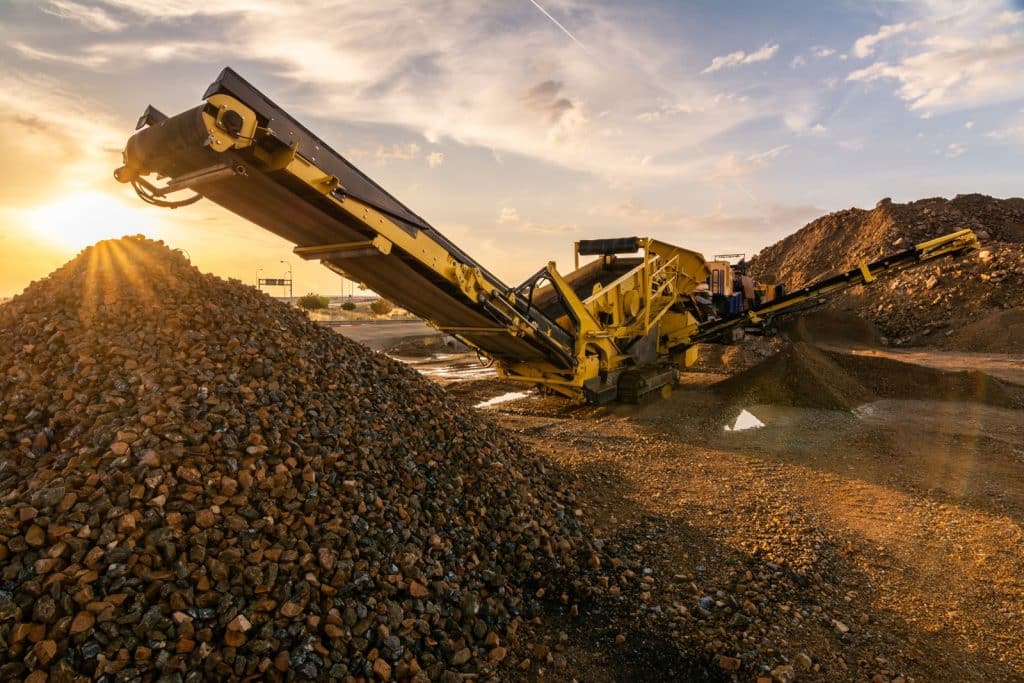This outdoor photograph appears to capture a mining site during the twilight hours, as the sun begins to set. Dominating the center of the image is a large, yellow machine fitted with two conveyor belts. These belts angle upward at approximately 45 degrees, stretching out towards both the left and right sides of the frame. Beneath these conveyor belts, there are sizable piles of rocks or pebbles, suggesting ongoing mining operations, potentially for gold. The sky occupies the top third of the rectangular photo, showcasing a light blue expanse with wispy white clouds. A glimpse of the sun can be seen on the upper left, casting an illuminating glow across the scene. To the left side of the image, there appears to be a road or highway adjacent to the mining equipment.